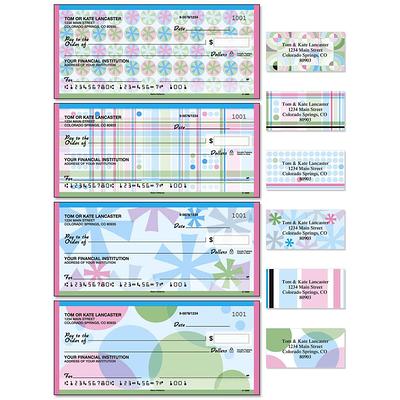The image depicts a collection of personalized checks and matching address labels, showcasing various colorful designs. At the top, there is a set of checks with a background resembling Christmas candies in different pastel colors, set against a pink and blue backdrop. Below, another set features a pattern of star-like items in blue, pink, and green hues. Further down, additional checks display a bubble pattern with the same color scheme. Each check includes fields for names, addresses, dates, and check numbers, with an example name like "Tom or Kate Lancaster" and check number 1001. To the right of the checks, there are six personalized address labels matching the check designs, illustrating how one's name and address would appear in the same pink, blue, and green pastel colors. The left side of the image provides an up-close view of the checks' layout, highlighting the lines and customization options. The overall theme is vibrant and floral, with predominant colors of pink, green, and blue.